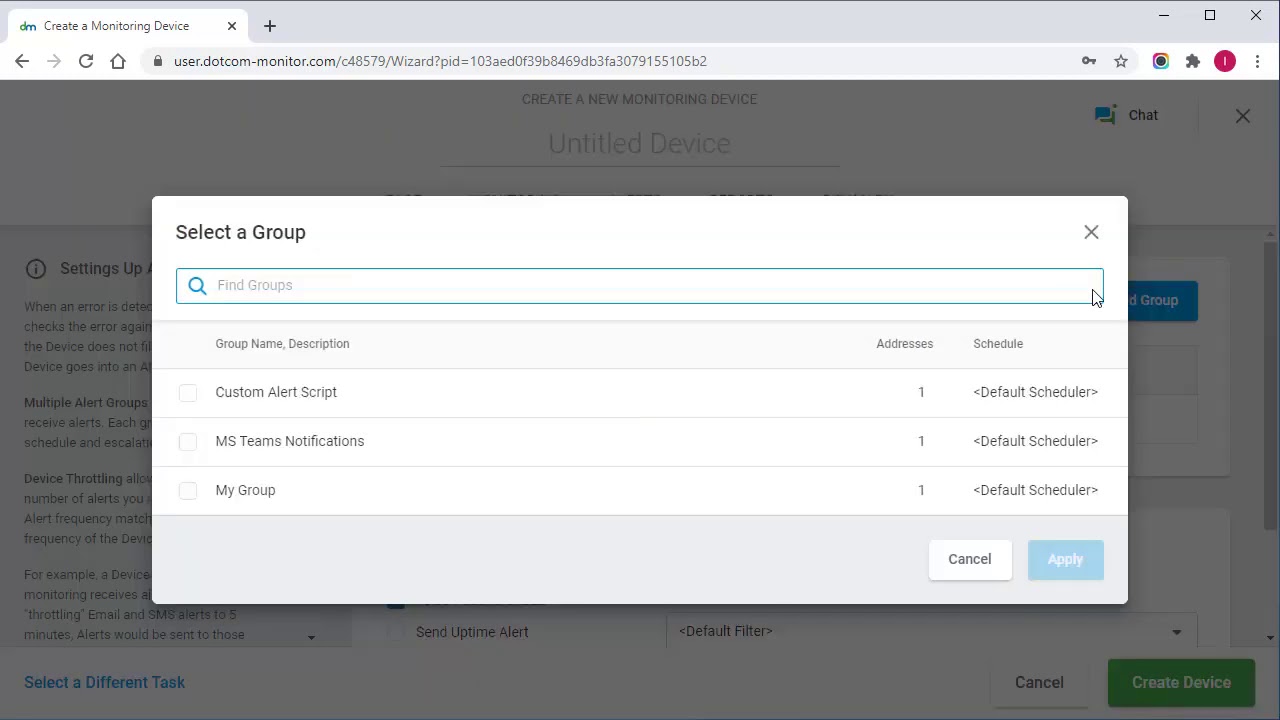**Detailed Caption:**

The image depicts the interface of a laptop screen focused on a browser tab titled "creating a monitoring device." At the top, the tab bar includes various navigation elements: to the right of the tab title is an "X" icon for closing the tab, and a button for adding a new tab. The tab title itself includes lowercase initials "DM" to the left. Below the tabs, there is a row with a back arrow, a refresh icon, a grayed-out forward arrow, and a home button. The URL bar displays "user.com," indicating the website in use. 

At the top right corner of the window, standard control icons are present: a minimize button (minus sign), a maximize button (square), and a close button ("X"). Beneath these controls, there are additional icons for key functions, including a favorites star among others.

In the main content area, there is a section titled "Create a New Monitoring Device," showing an "Untitled Device." To the right, buttons for chat support and closing the section appear, followed by settings options and an "Add a Group" link highlighted in blue. Below this, another section offers a "Select a Different Task" link in blue, followed by a "Cancel" button in white and a "Create a Device" button in green.

In the central part of the screen, a "Select a Group" dialog box is open. It contains a search bar labeled "Find Group" and columns for group name, description, custom alert script, and MS Team notification of "My Group," with none of the options currently selected. The section also includes addresses labeled as 'all one' and a schedule column. At the bottom of this dialog box, "Cancel" and "Apply" buttons are available for user interaction.